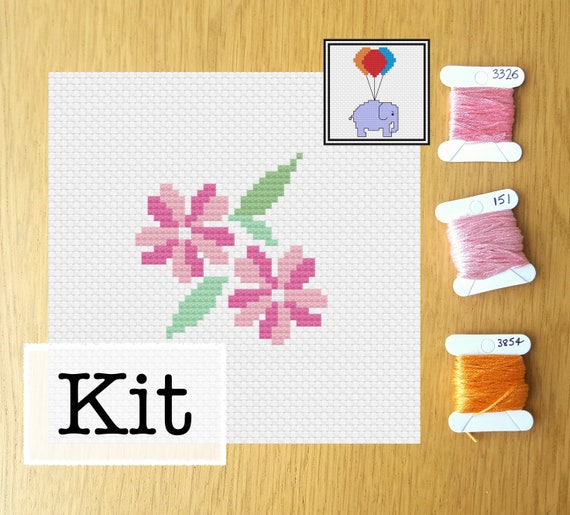The image depicts a detailed embroidery kit sitting atop a light blonde wooden table. At the center of the image, there's a square of off-white fabric showcasing a template for two flowers with variegated pink petals and oblong, pointy green leaves. To the right of this fabric template are three skeins of embroidery floss, each wound around cardboard holders marked with numbers: the top, a dark pink labeled 3326, the middle, a lighter pink labeled 151, and the bottom, a bright orange labeled 3854. Additionally, the kit previews a smaller design featuring a gray elephant being carried by three balloons—one blue, one red, and one orange. In the bottom left corner, the word "KIT" is prominently displayed inside a rectangle, reinforcing the nature of the product.